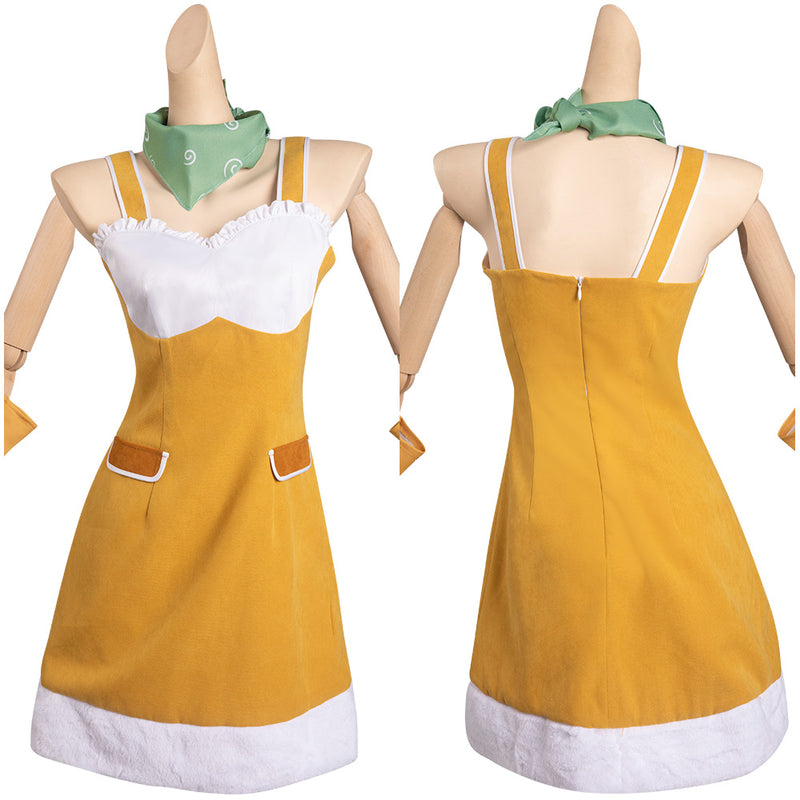The photograph features two slender, headless mannequins with articulated arms, showcasing a vibrant summer shift dress from both the front and the back perspectives. Each mannequin sports a neatly folded, mint-green neckerchief with white spirals, adding a touch of elegance to the ensemble. The dress is predominantly mustard yellow, with a form-fitting design that tapers at the waist. The upper part of the dress has a distinctive white brassiere-like highlight, reminiscent of a bikini top, and the dress itself features white borders on the shoulder straps and a white hem at the bottom. 

On the front of the dress, there are two mustard-colored, flat rectangular pockets with white outlines, one on each side, providing a subtle yet practical detail. The back of the dress maintains the mustard yellow color with a central zipper running from top to bottom and has no additional pockets or dark brown highlights. Though partially obscured, it appears that the mannequins may be wearing gloves.